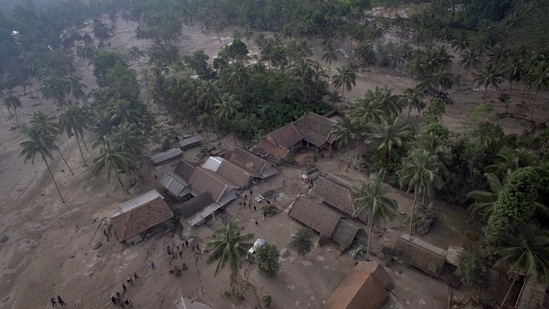The image portrays an aerial view of a small village nestled on a sandy, dirt-paved area surrounded by trees, including numerous palm trees suggestive of a tropical setting. The village appears to be in a mountainous region, given the arrangement of the trees and structures. The houses dominate the center of the image, extending towards the bottom right corner, each marooned in a pool of brown, floodwater, indicating that the area has recently experienced heavy rains and likely a massive flood. The river, responsible for the overflow, is seen at the top of the image. Some houses exhibit subtle details, possibly including thatched roofs or other distinguishing features. No readable text is visible in the picture. The overall color palette includes green from the trees, white and gray from the houses, and a brownish tone from the water and sandy roads.